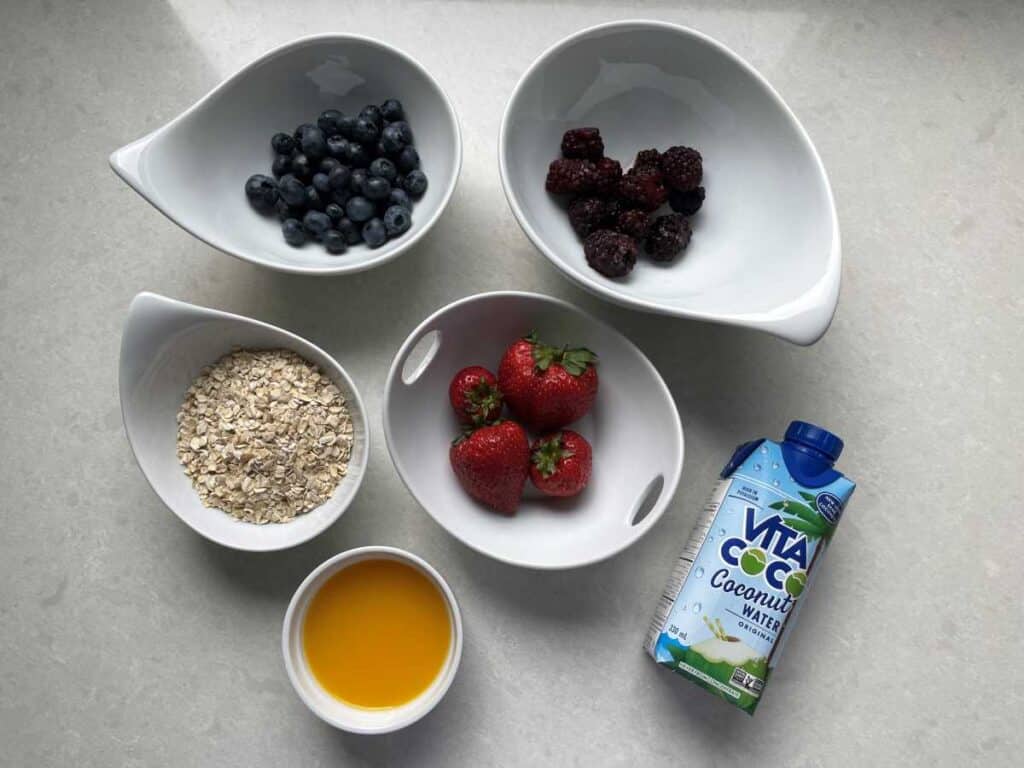A vibrant and healthy assortment of foods is artfully arranged on a white, stone-like surface in this overhead shot. The composition features five uniquely shaped bowls, including a circular one, an oval one, and three teardrop-shaped bowls. The bowls contain a mix of colorful ingredients: blueberries, blackberries, strawberries, oats, and an orange-colored dipping sauce. The blueberries are particularly abundant. Adjacent to the bowls is a bottle of Vita Coco coconut water, labeled "Fight the Cocoa," adorned with illustrations of palm trees and coconuts. The objects are casually clustered together without a specific pattern, and the photo’s setting remains ambiguous, capturing the vibrant hues of blue, red, dark purple, black, tan, beige, orange, and green against the neutral background.